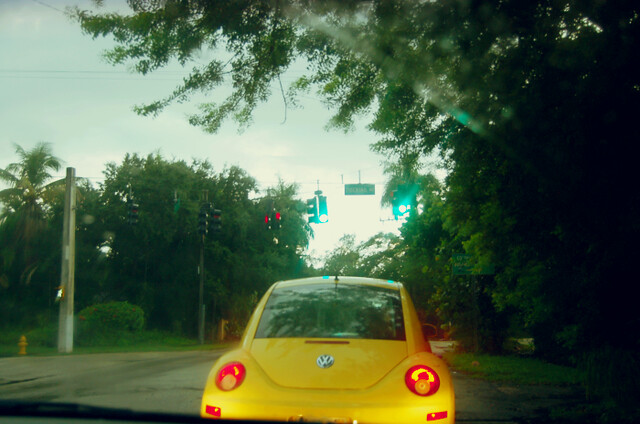In this outdoor image, a bright yellow Volkswagen buggy is prominently displayed. The vehicle's taillights, two vivid red lights on either side, are illuminated, suggesting it is either parked or preparing to move. Positioned above the buggy is a sizeable rearview mirror reflecting an indistinct scene. Surrounding the buggy, the environment is rich with details: lush green leaves frame both the left and right sides of the image, indicating a possibly verdant area. The sky overhead is overcast with numerous gray clouds. The ground beneath the buggy is paved with asphalt, and to the left, there's a metal pole standing sentinel. Nearby, traffic lights indicate directional movement; the lights are red for left and right turns, while a green signal points straight ahead. Additionally, there's a green road sign providing directions, contrasting with another green traffic light in close proximity. Despite the array of signals, the buggy remains stationary, with its crimson taillights punctuating the scene.